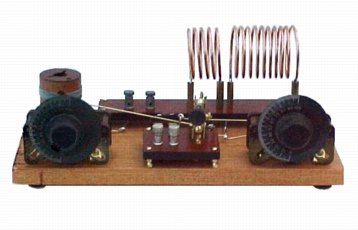The image depicts an antique machine, likely from the early 1900s to 1920s, mounted on a rectangular wooden board with small rubber feet at each corner. The background is entirely white. In the front, two identical round black dials with illegible white numbers are positioned on the left and right sides, resembling speakers or radio components. Between them, a central console features several knobs and antenna-like metal columns, including two smaller silver ones and a brass one with wires extending to the right-hand dial. Towards the back, a large coil of wire loops prominently on the right-hand side, mounted on another darker wooden panel. Additionally, behind the left dial, there is a round wooden object wrapped with blue string. The overall complexity and array of coiled wires and metal columns suggest it might be the inner workings of an early radio or telegraph machine. The photograph lacks textual labels, making the exact identification of the device challenging.